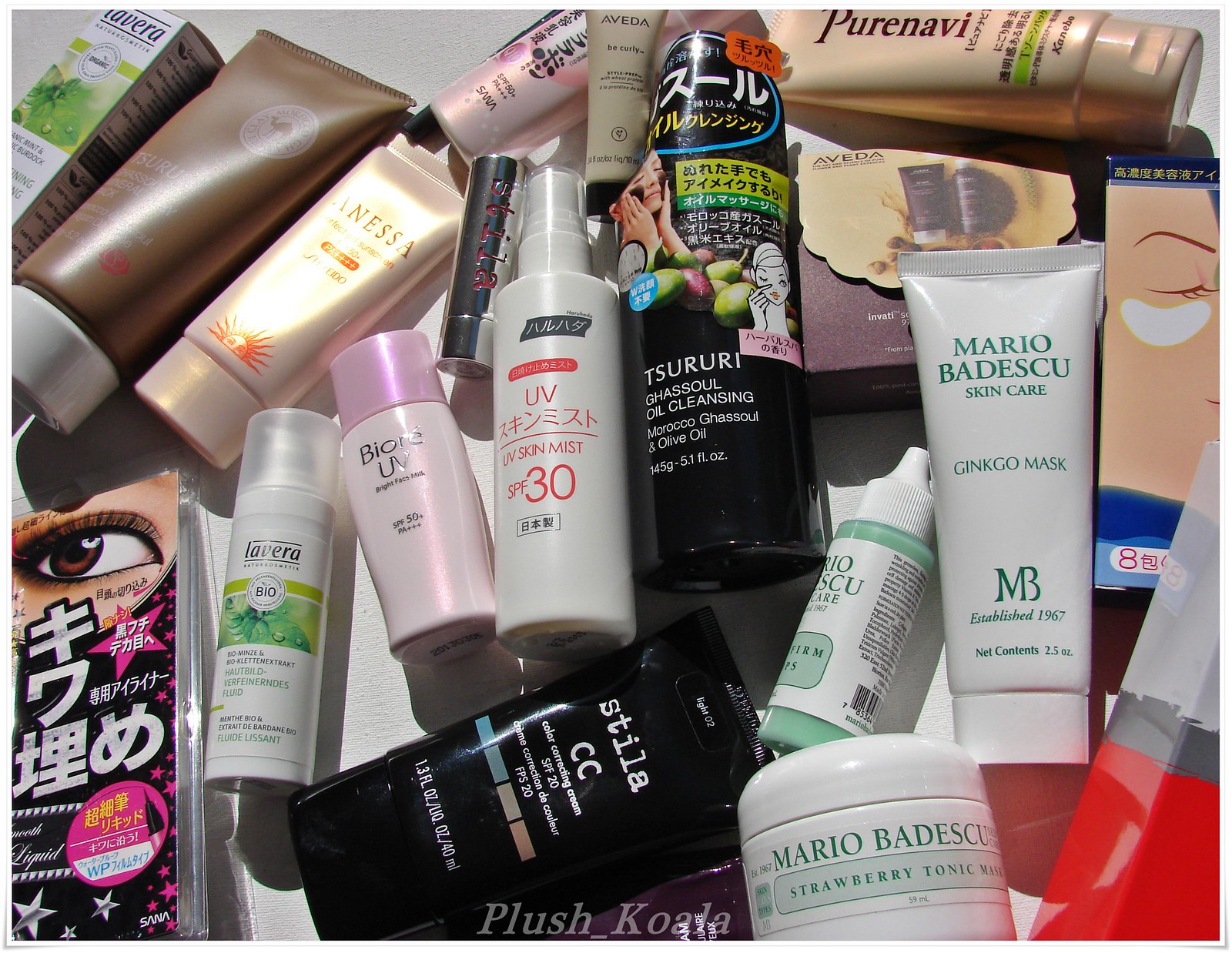This detailed image showcases a carefully arranged collection of skincare and makeup products. Starting at the bottom left, there's a makeup package adorned with Asian-style text, featuring a pink circle with yellow text, a pink star with white text, cursive white words, and an image of a brown eye. To its right sits a white bottle with a logo of a green plant at its center. Further right, another white bottle sports a purple cap, followed by a white bottle with red text.

Below these, a black bottle lies on its side, next to a small container labeled "Mario Badescu Strawberry Tonic." To its right is a product with a distinctive half-red, half-gray design. Above these items is a tub labeled "Mario Badescu Skincare Wrinkle Mask," featuring the initials "MB" in green. Adjacent to this is a blue package and to its left, a small green and white bottle. Above this, a black bottle is partially visible.

Additionally, there are several small lipstick containers in gray, a gray bottle with orange designs brightly illuminated by light, and a brown bottle positioned at the top left next to a rectangular package. A pink hue caps off the collection at the very top. The entire composition is set against a subtly lit light gray background.